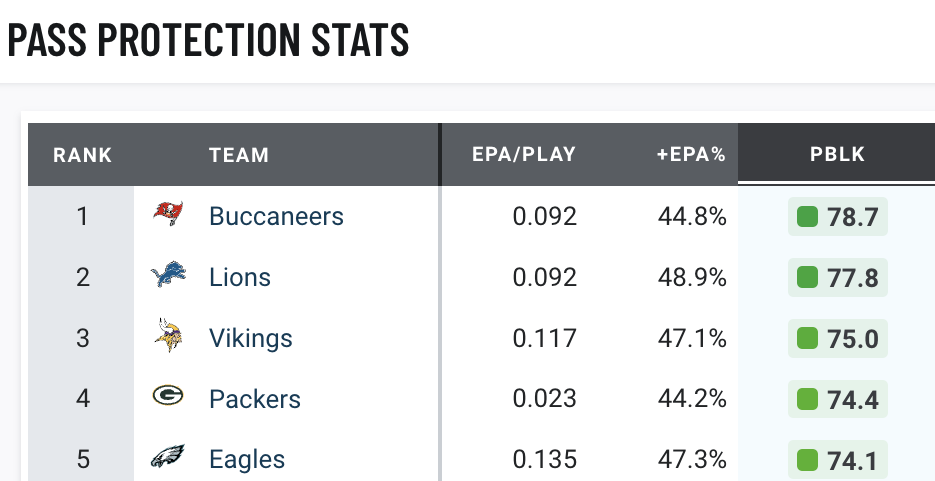A cropped screenshot from an app displays the past protection stats for various NFL teams, ranked from 1 to 5. The rankings and corresponding teams are:

1. Buccaneers - Featuring a pirate flag logo
2. Lions - Represented by a blue lion logo
3. Vikings - Depicted with a logo of a Viking head with blonde hair and a horned helmet
4. Packers - Identified by a "G" logo
5. Eagles - Illustrated with a stylized eagle head

The stats table includes the following metrics: EPA (Expected Points Added), EPA% (EPA Percentage), Plus EPA%, and PBLK (Pass Block Win Rate). The specific values for each team are as follows:

- Buccaneers: 
  - EPA: 0.092
  - EPA%: 44.8%
  - Plus EPA%: 78.7

- Lions:
  - EPA: 0.092
  - EPA%: 48.9%
  - Plus EPA%: 77.8

- Vikings:
  - EPA: 0.117
  - EPA%: 47.1%
  - Plus EPA%: 75.0

- Packers:
  - EPA: 0.023
  - EPA%: 44.2%
  - Plus EPA%: 74.4

- Eagles:
  - EPA: 0.135
  - EPA%: 47.3%
  - Plus EPA%: 74.1